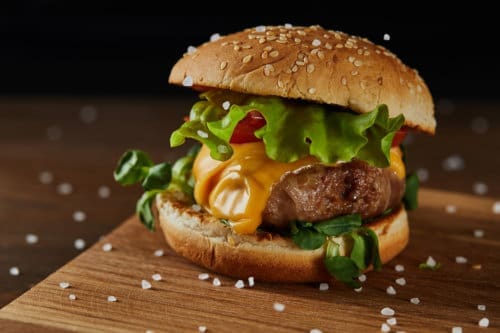This detailed photograph captures a close-up of a small, thick cheeseburger, likely a slider, resting on a wooden cutting board which is sprinkled with large white granules of rock salt. The toasted, sesame-seeded bun, possibly whole wheat, crowns the burger. The patty, made of ground beef, is generously topped with melted orange cheese, possibly cheddar or American. Beneath and above the cheese are layers of fresh, curly romaine lettuce and a slice of ripe red tomato. The background of the image is a darker wooden table, blurring out to a near-black hue, with scattered specks of salt and seeds enhancing the rustic aesthetic of the presentation.